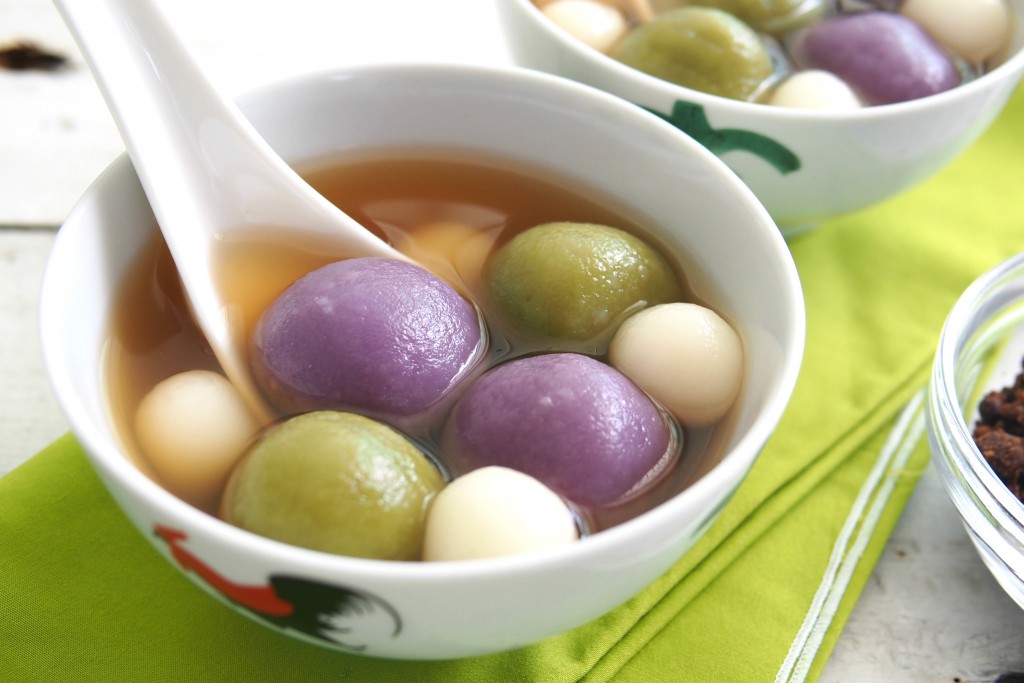This color photograph captures two white ceramic bowls positioned next to each other on a green tablecloth with white stripes, atop a white-painted wooden table. The bowl in the lower right is fully visible and contains a white ceramic spoon. These bowls feature distinct designs: the lower one has a red and black rooster, while the upper bowl includes a green design partially visible. Both bowls are filled with a traditional Asian dish, likely sesame ball or mochi ball soup, with a yellowish-brown broth resembling the color of tea. Floating within the broth are several glutinous rice balls in various colors: two purple, two green, and four smaller white balls. A partially seen third bowl with a different food item can also be observed in the background.